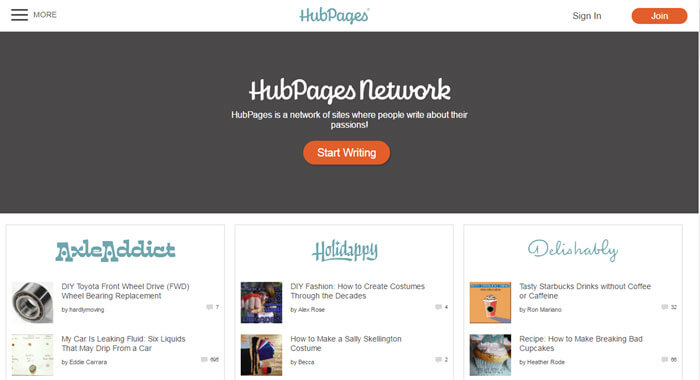The image showcases the homepage of Hub Pages, a network of sites dedicated to writers and bloggers. The dominant feature of the page is a soft black background with the text "Hub Pages Network" stylized in cursive font. 

At the center of the screen, there is a large, inviting orange button labeled “Start Writing,” encouraging users to begin contributing their content. Above this, the top navigation bar includes a “More” button represented by a hamburger icon (three horizontal lines), along with “Sign In” and “Join” buttons for user authentication and registration.

Directly below the black header area, the page transitions into a white section displaying a selection of various articles. These articles are from the diverse categories within the Hub Pages network, each seemingly tailored to specific interests. For instance, the “AxleAddict” section contains posts such as "DIY Toyota Front Wheel Drive Wheel Bearing Replacement" and "My Car is Leaking Fluid: Six Liquids That May Drip from Your Car," indicating a focus on automotive DIY content. 

Additionally, sections like “Holidappy” feature more DIY topics, while “Delishably” provides content related to food, as suggested by its name. The overall image serves as a snapshot of the Hub Pages platform, highlighting its role as a space for enthusiasts to share their knowledge and passions across a variety of subjects.